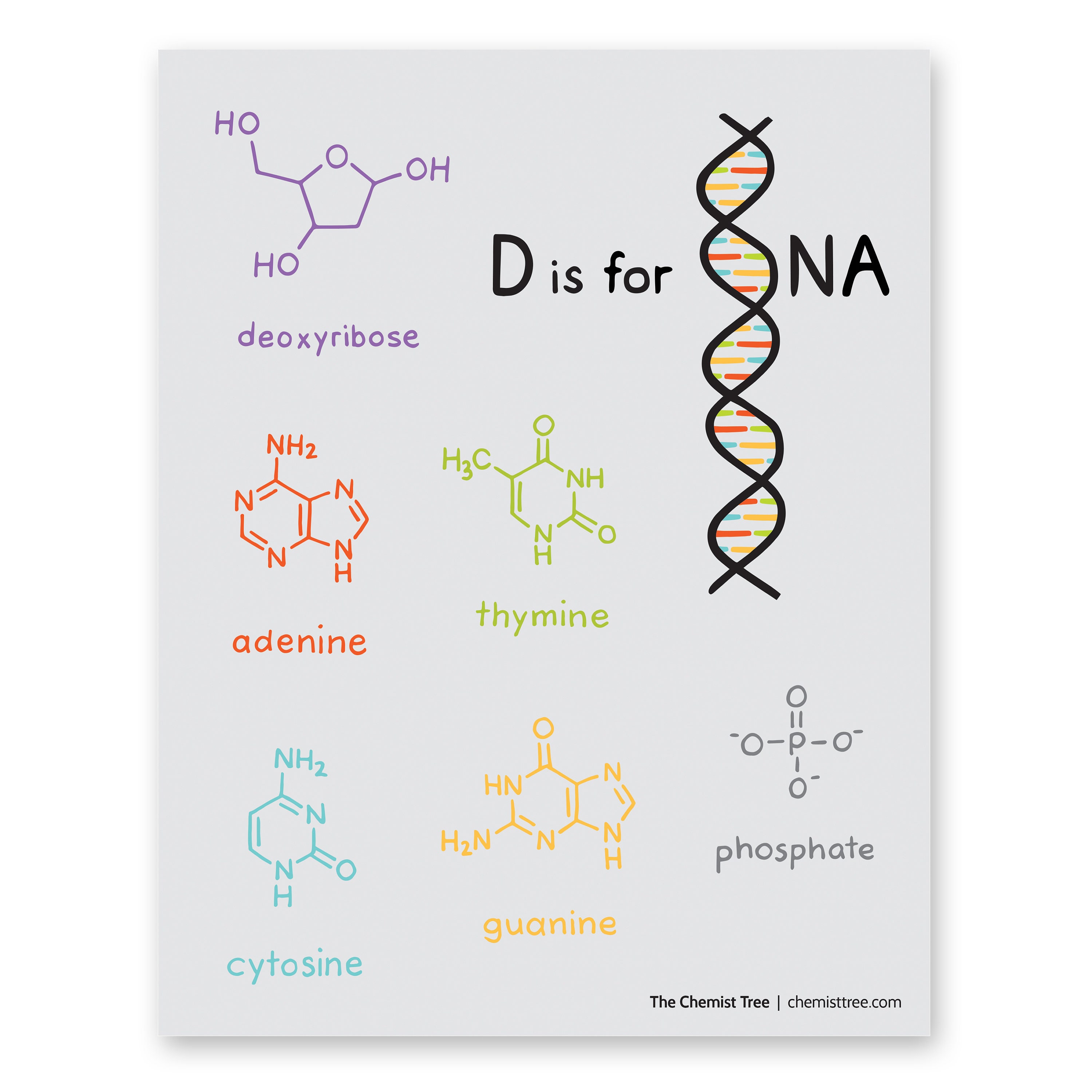This image is a detailed, hand-drawn-style illustration set on a white, rectangular background, resembling a page from a textbook or a framed artwork. The central focus is on various molecular structures associated with DNA, each uniquely colored for easy differentiation. In the top right corner, the phrase "D is for DNA" is cleverly depicted with a DNA double helix symbol forming the letter "D." The bottom right corner is marked with a black watermark that reads "the chemist tree, chemistry.com."

The diagram includes:
- Deoxyribose in purple, visualized as a hexagon or pentagon connected by HO, OH, and O groups.
- Adenine in red.
- Thymine in green.
- Cytosine in blue.
- Guanine in yellow.
- Phosphate in gray.

These molecules are spaced out across the image, each labeled with its name and structure, and are designed in various bright colors to enhance visual appeal. The poster, with its educational yet artistic portrayal, appears to be an advertisement for an item available for purchase, aimed at those interested in the fundamentals of chemistry and DNA.